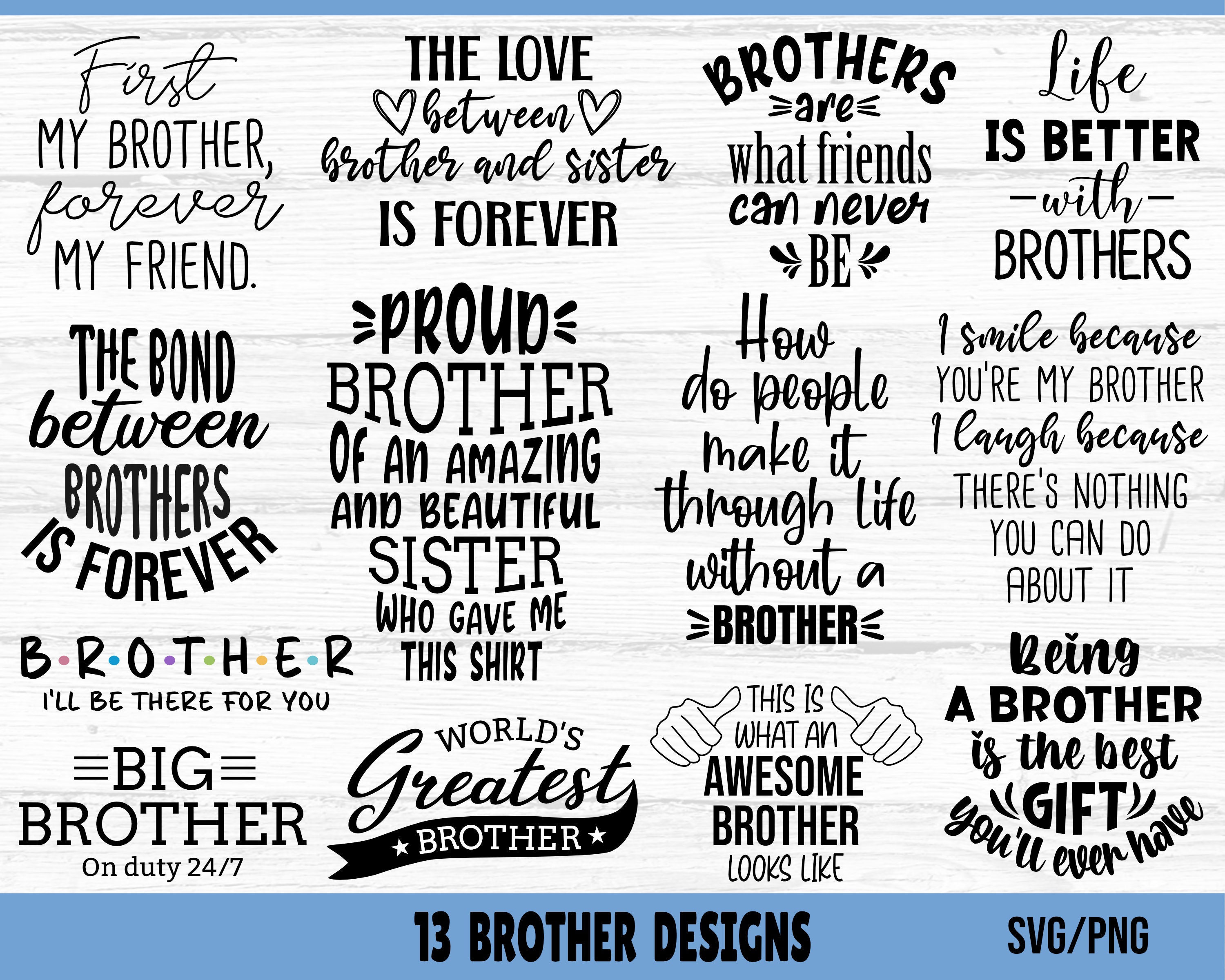The image showcases a collection of 13 brother-themed designs for various products, such as shirts or mugs, labeled at the bottom with "13 Brother Designs" in a blue banner followed by "SVG/PNG" file formats. Each design features unique slogans celebrating brotherhood, with phrases like "First my brother, forever my friend," "The bond between brothers is forever," "Big brother on duty 24/7," and "Proud brother of an amazing and beautiful sister who gave me this shirt." Other phrases include "World's greatest brother," "Brothers are what friends can never be," "How do people make it through life without a brother?" and "This is what an awesome brother looks like." One design humorously reads "I smile because you're my brother. I laugh because there's nothing you can do about it." Another mentions, "Life is better with brothers," and "Being a brother is the best gift you'll ever have." Some designs incorporate simple line illustrations, such as thumbs pointing inward or phrase stylizations, like the "Brother, I'll be there for you" in the style of the Friends TV show logo. The fonts vary in format, ranging from bold to stylized lettering, adding to the visual diversity of the designs.